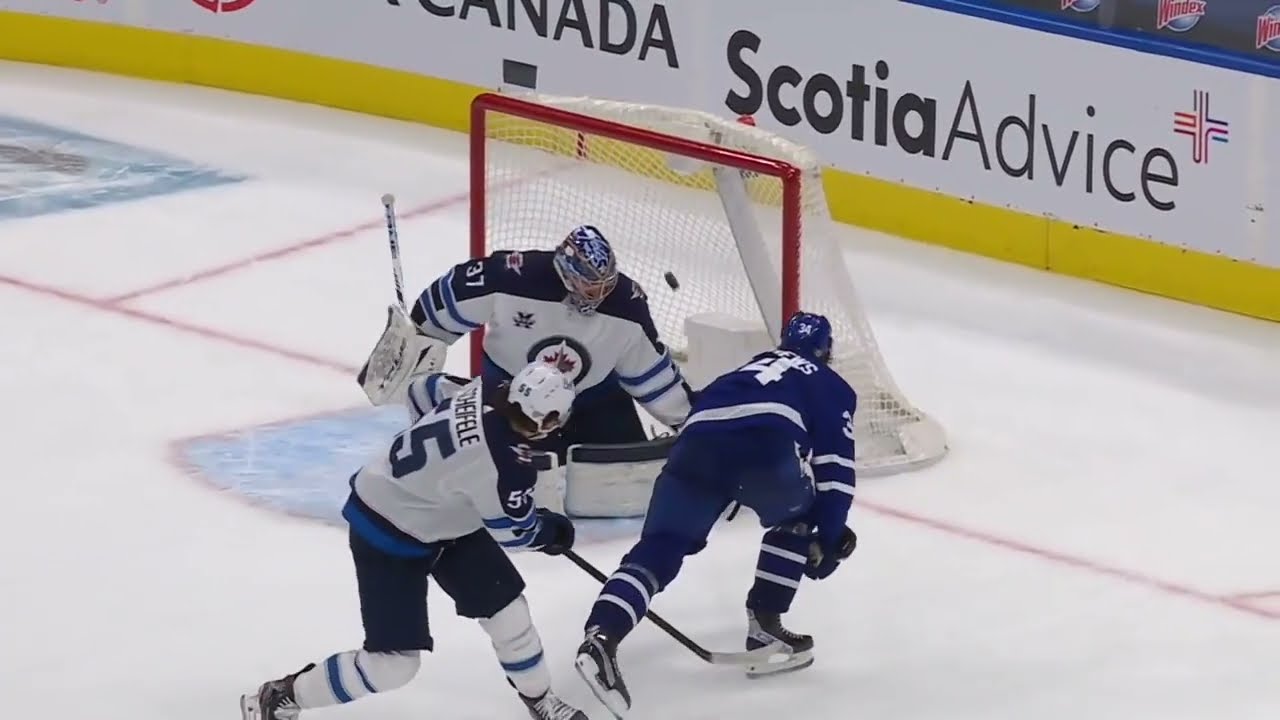The image depicts a tense indoor ice hockey game with three players prominently in focus at the center. Two players, positioned to the left, are wearing matching white jerseys with black shoulders and black pants. The player to the right is clad in a royal blue jersey with white stripes. They are all heavily equipped, including helmets and skates. Behind the players, a red-framed goal with a white net stands out against the white, slightly scuffed ice with some blue and red lines permeating through. The background wall is white with a yellow strip at the bottom edge, prominently displaying the words "Canada," "Scotia Advice," and a must-see, a red and blue cross-shaped logo. The familiar Nike logo is also discernible, along with several imprints of “Windex,” indicating sponsorship logos lining the rink.